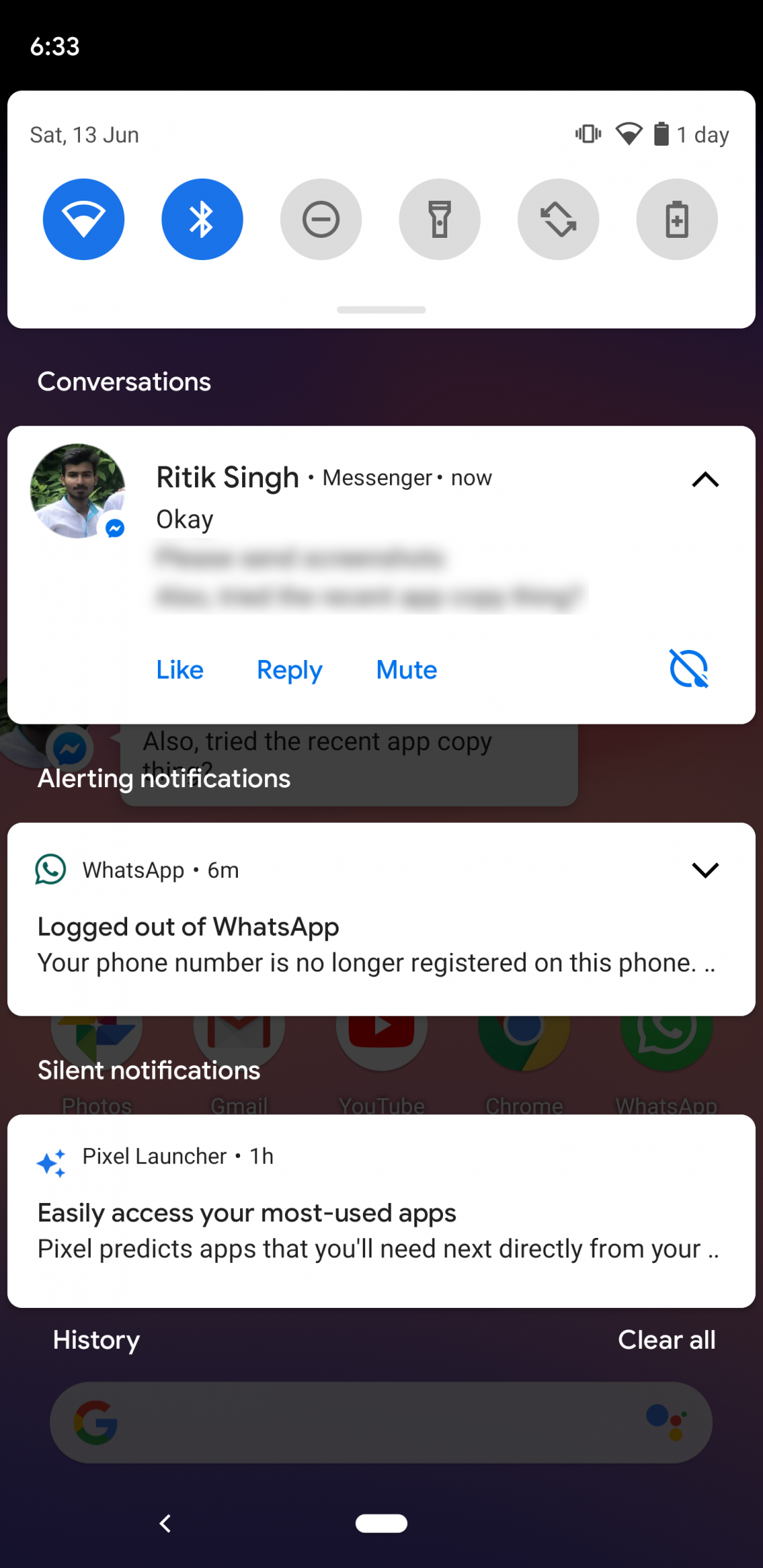In the image, at the top left corner, the current time displayed is 6:33. Beneath this is a small boxed area containing six icons. The first icon on the left appears to be a WiFi symbol with two bars filled, indicating a moderate connection. Next to it is the Bluetooth symbol, followed by a circular icon with a dash through the middle. The fourth icon resembles a flashlight, and the fifth icon consists of two arrows forming a rectangular shape, possibly representing screen rotation. The last icon is a battery symbol. Within this boxed area, "Saturday, 13 June" is displayed at the top left, and at the top right are small icons showing a vibrating phone, WiFi signal strength, and a nearly full battery.

Below this box, there is a section titled "Conversations," featuring another boxed area with a person's name, Rateek Singh, to the left, and "Messenger now" to the right. Below this is a blurred-out message that Rateek wrote. At the bottom of this box are options in blue text: "Like," "Reply," and "Mute."

The lower half of the image contains two more boxes. The first box is labeled "Alerting Notifications," while the box below it is titled "Silent Notifications."